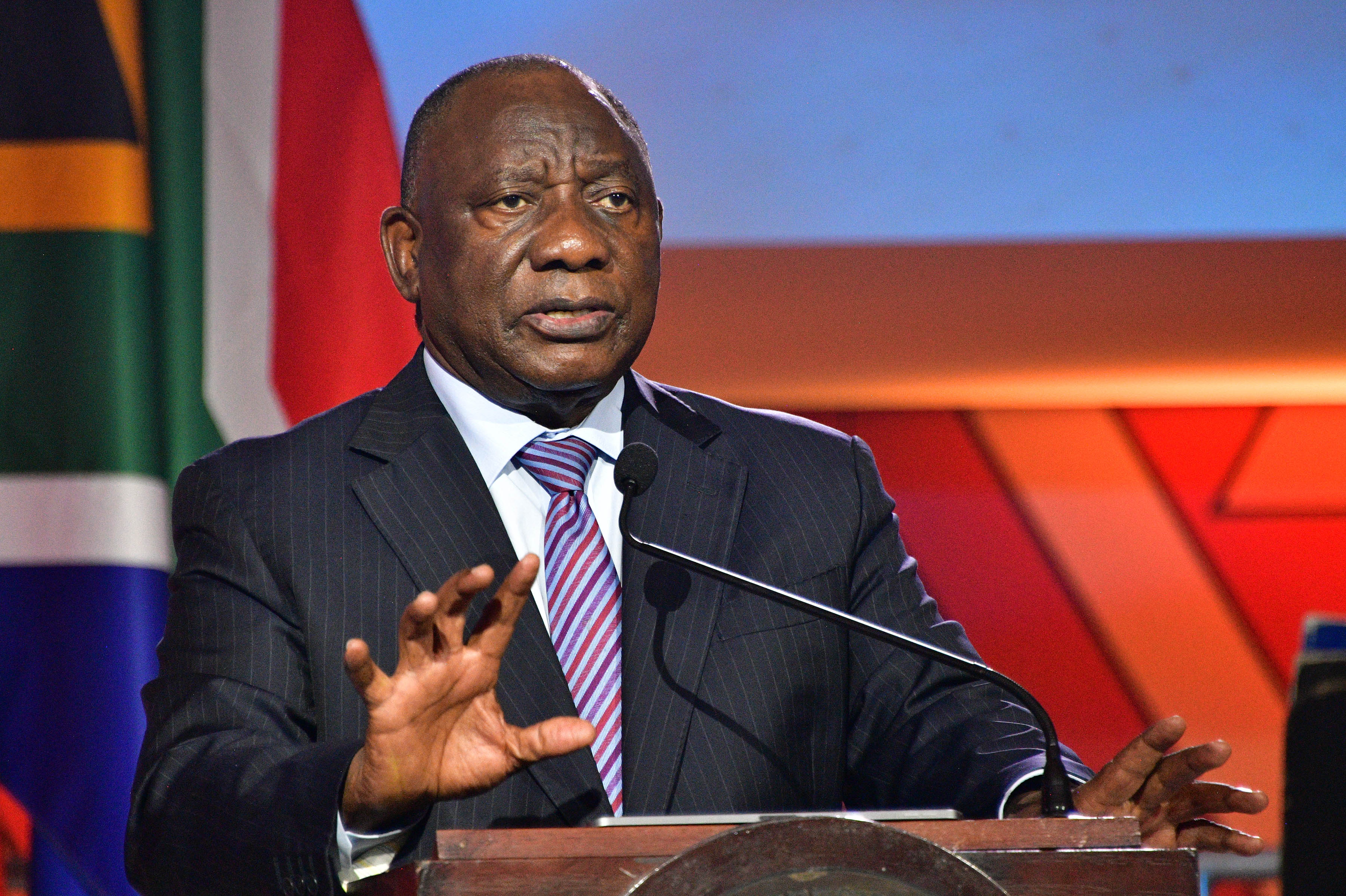This image features Cyril Ramaphosa, President of South Africa, standing solemnly at a wooden podium equipped with a microphone. He is dressed in a dark blue pinstripe suit, complemented by a button-down collared shirt, and a tie adorned with diagonal stripes in shades of blue, red, and purple. His robust round face is marked by a stern expression, with his forehead slightly wrinkled, and he directs his gaze just off to the right.

Ramaphosa's right hand is raised, palm visible, as if he is emphasizing a point, while his left hand rests open on the podium. Behind him, a vivid backdrop features a combination of colors including yellow, green, red, blue, and brown. A flag with possible colors of red, white, green, and blue is also visible among the vibrant hues, suggesting a ceremonial or formal setting. The blue background further accentuates Ramaphosa's poised figure as he addresses his audience.